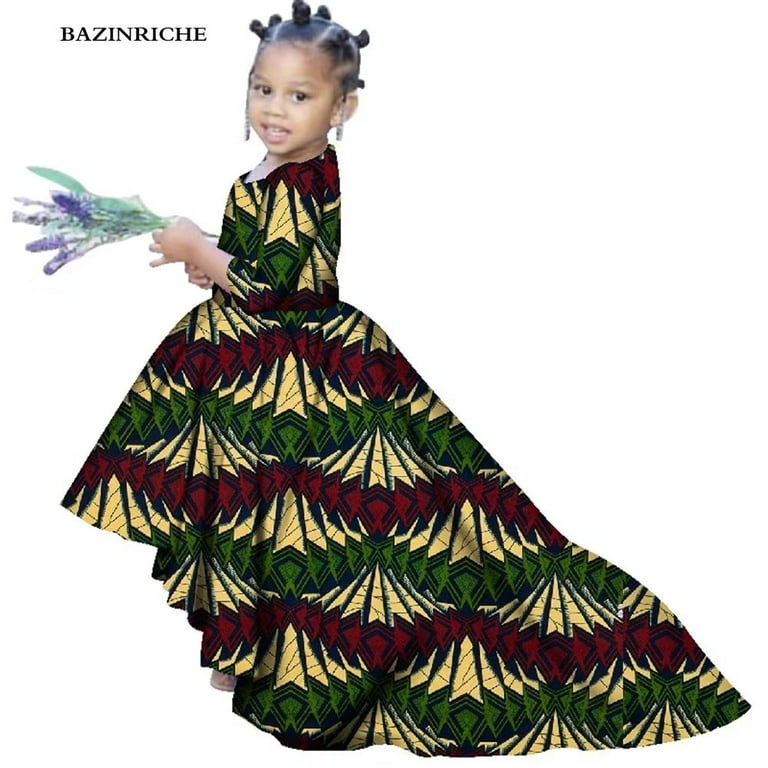This image features a young, light-skinned African-American girl, approximately five years old, dressed in a vibrant, colorful long dress that flows to the floor and has a slight train. The dress is adorned with geometric patterns, including diamonds and triangles in hues of red, yellow, and green. She holds a small bouquet of flowers with green stems and purple tips, although the specific type of flowers is unclear. Her hair is styled in six visible buns, each decorated with tiny enamel clips, and she wears a gentle half-smile, showcasing her big brown eyes. Positioned at the top left of the image, the text "Bazinriche" (B-A-Z-I-N-R-I-C-H-E) appears in black font, possibly indicating the brand or designer of the dress.